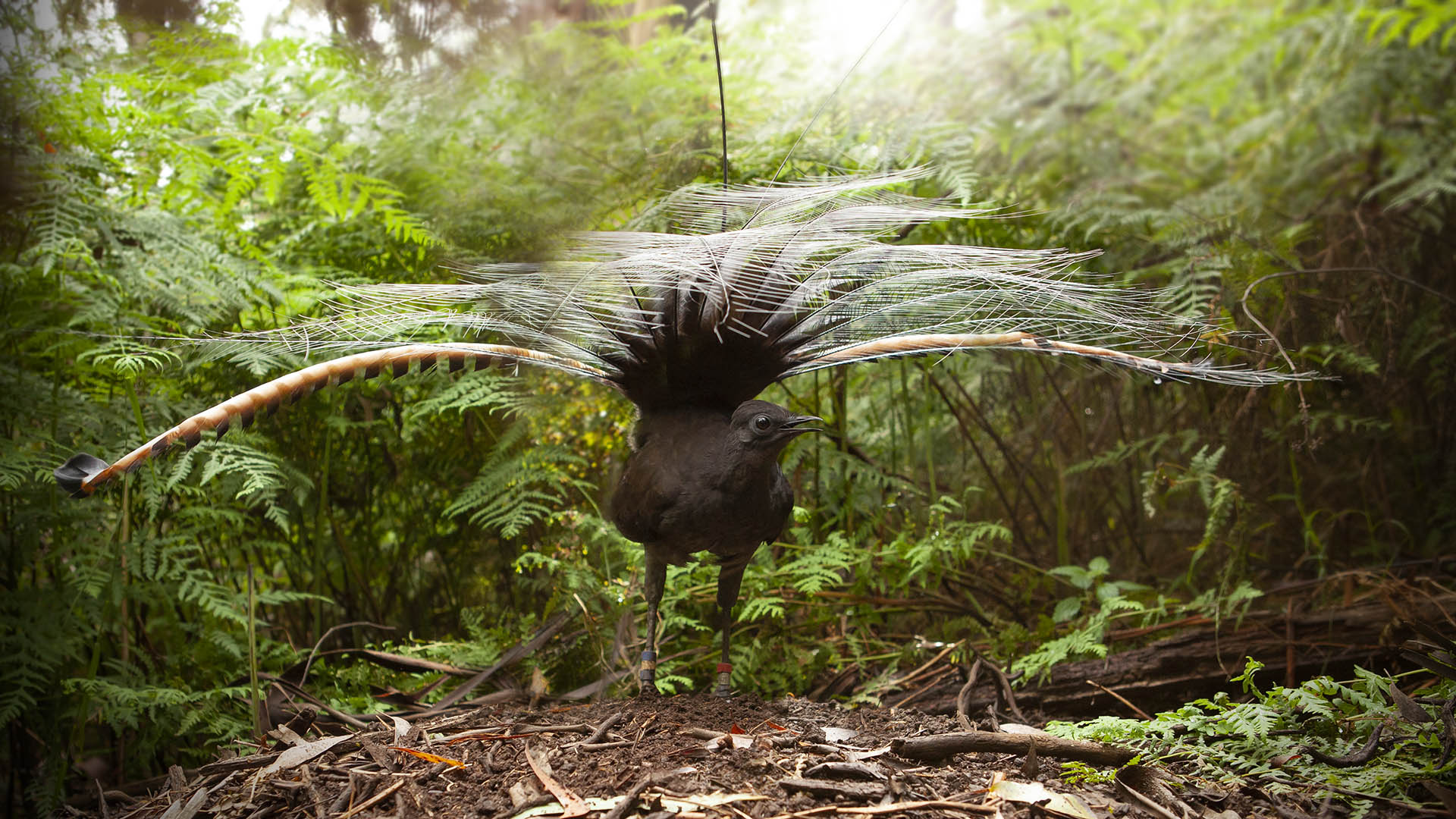In a vividly green forest clearing, a mysterious, sizable bird with an uncanny resemblance to a peacock stands out amidst a rich carpet of dead leaves, branches, soil, and mulch. This enigmatic creature, which appears to be AI-generated due to its overly smooth texture and unusual features, captures attention with its impressive wingspan. The bird has large, spider web-like wings adorned with hints of white, which are blurred in motion as they stretch towards the ground. Its body is predominantly black, contrasting sharply with its unique tail that fans out like a peacock's but consists of delicate, white feather strands forming intricate, web-like patterns. Surrounding the bird are lush green ferns, bushes, and various other plants, creating a vibrant backdrop bathed in streaming sunlight that filters through, adding a glowing, almost ethereal effect to the scene. The bird, with its open beak, looks towards the right, standing majestically as it dominates the forest floor, surrounded by the dense plant life that obscures the taller trees in the background.